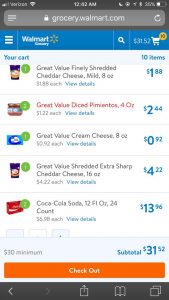The image showcases a smartphone screen displaying the Walmart Grocery website. At the very top of the screen, the status bar indicates the device is linked to Verizon, displaying signal strength and the time as 12:42 a.m. To the far right, a series of icons, including a battery icon showing less than half charge, are visible. 

Below the status bar, there's a gray URL bar that reads "grocery.walmart.com." Adjacent to the URL are a refresh icon and a menu icon with three horizontal lines. Underneath the URL bar, a blue navigation bar prominently features the Walmart Grocery logo, accompanied by a search icon and a cart icon showing a total of $31.52 worth of items in the cart.

The main section of the screen lists the items currently in the cart, detailing each item's quantity and total cost. Items listed include Great Value Diced Pimentos (4 ounces), which is specifically highlighted in red, while other items are listed in black. The cumulative cart total is displayed at the bottom as $31.52, noted against a $30 minimum purchase requirement. An orange "Checkout" button is positioned towards the bottom of the screen. All item prices and the subtotal are highlighted in blue, ensuring clarity on the total cost and individual item expenses.